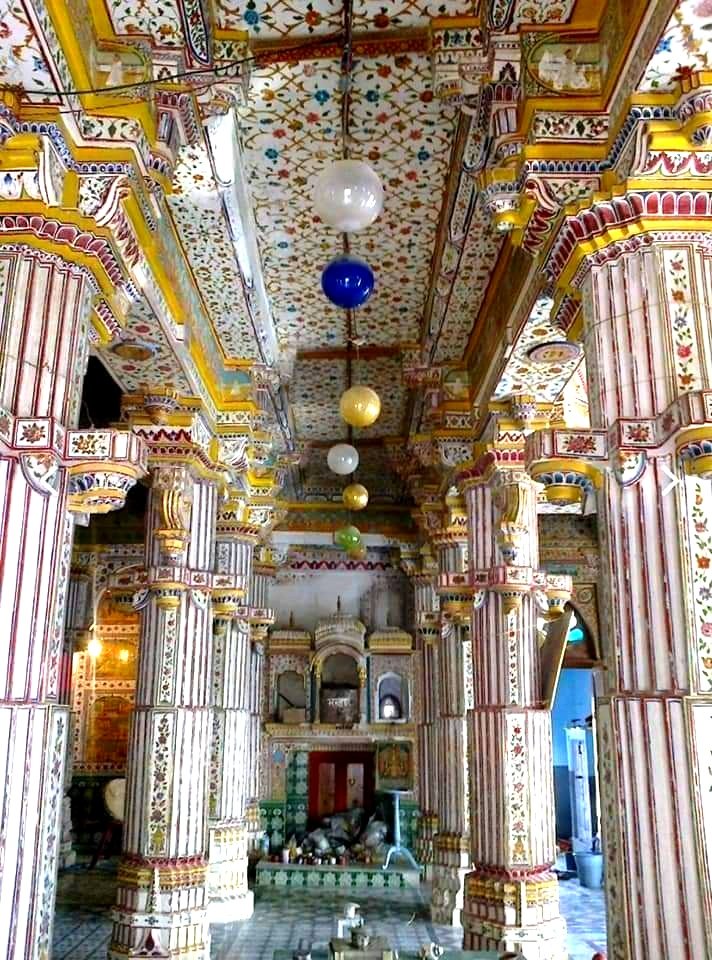The image depicts the interior of an ornately decorated older building, suggestive of a temple or a place of reverence, likely situated in Asia. The structure boasts a vibrant and colorful design, with an array of architectural details that capture the eye. Central to the scene are multiple concrete columns, eight in total, arranged symmetrically—four on each side. These columns are adorned with red and white pinstripes and gold motifs, and feature intricate three-dimensional moldings at their tops, embellished with small red arch shapes and yellow stripes.

The high ceiling is richly decorated with floral motifs in red, orange, gold, and blue, adding to the elaborate aesthetic. Hanging from the ceiling are glass or ceramic globes in colors of white, blue, yellow, green, and possibly some other bright shades, adding to the allure of the space. The floor consists of green tiles arranged in a captivating pattern, contributing to the overall grandeur of the interior. The background reveals compartments or alcoves which might be used for displays or as part of the reverence space, all of which are integrated into this fantastically detailed piece of architecture.